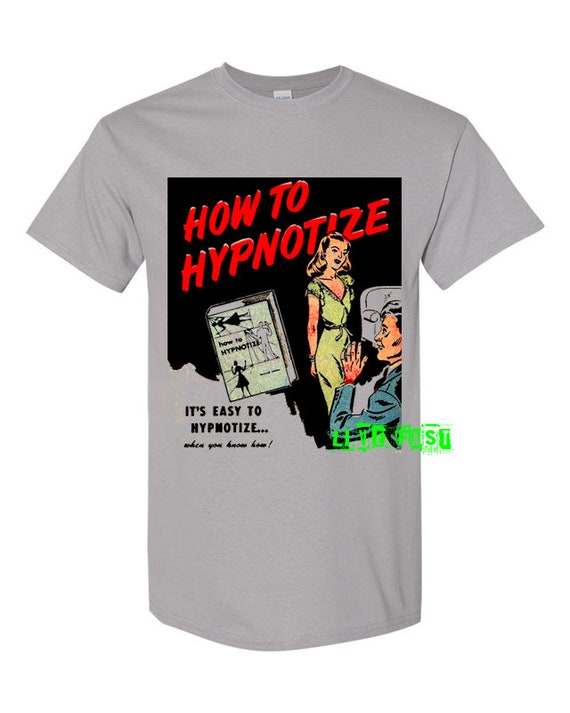This photograph features a light gray short-sleeved t-shirt with a custom design printed on it, set against a white background. Centered on the shirt is a square graphic with a black background, giving it a vintage 1940s-1950s comic book feel. The design prominently features the phrase "How to Hypnotize" in bright red text diagonally across the top. Below this, additional text states "It's easy to hypnotize, when you know how." 

To the right of the text, there is an image of a woman in a light green dress, reminiscent of 1940s American fashion. With shoulder-length blonde hair, she is looking down at a man seated in front of her. The man, dressed in a blue suit jacket, is gazing up at her intently. Beside the woman, there's a depiction of a green book titled "How to Hypnotize." The design extends to the lower right corner of the shirt, adding a subtle complexity to the overall appearance.

Despite the intricacies and vintage appeal of the design, the overall aesthetic has been poorly received by some viewers.